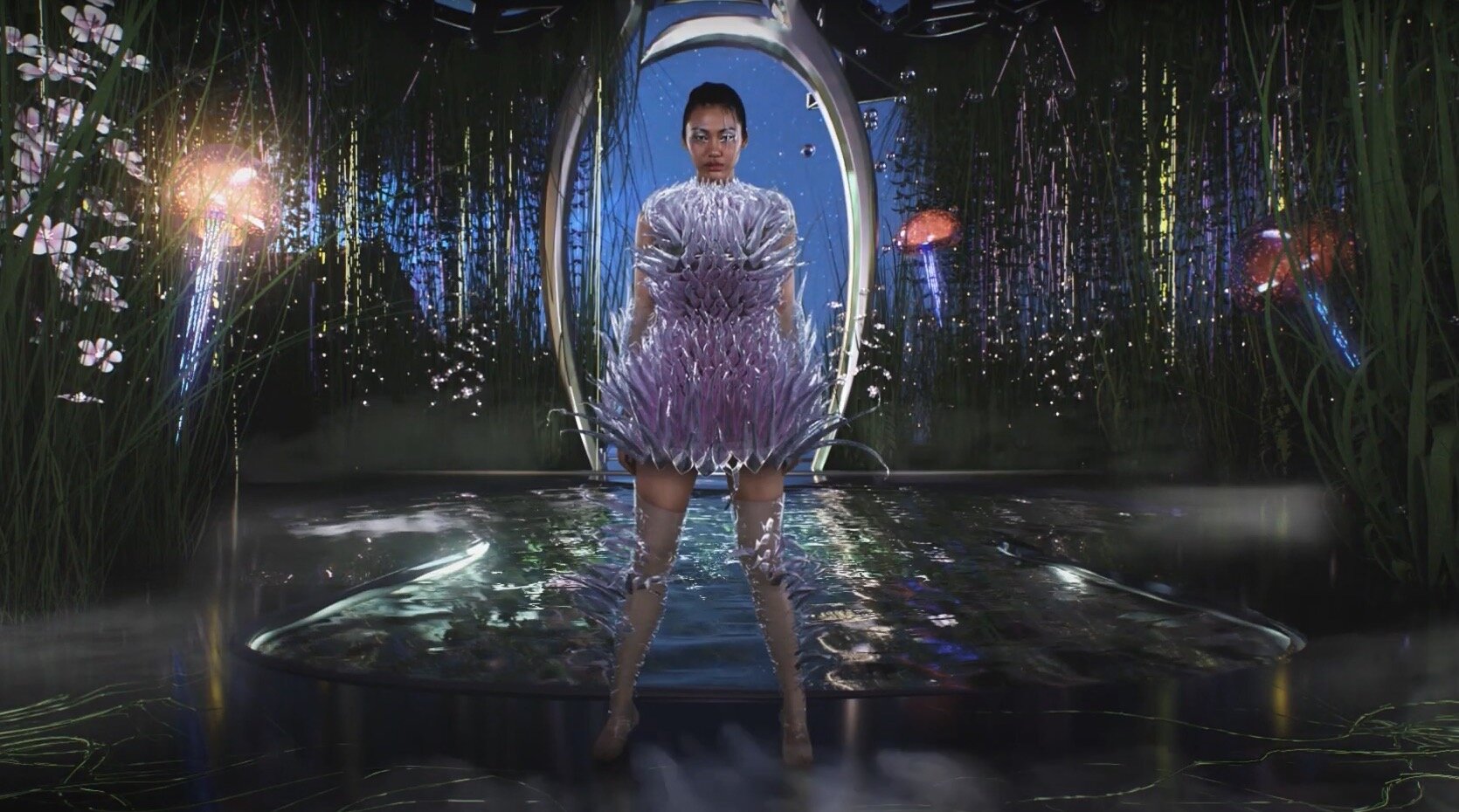The image portrays a striking, highly edited professional photograph set in a fantastical, futuristic garden scene. At the center stands an Asian woman, possibly in her late teens or early twenties, with a fierce expression. Her dark brown-black hair is styled in an elegant updo, held within a silver archway that frames her head and upper body. She wears a short, pale lilac dress with a textured, coral- or flower-like design, spiky tentacles extending from it, and appears to be standing on high heels, though they are partially obscured. The woman's legs are spread slightly, defining her triangular stance, and she stands knee-deep in a large reflective puddle. 

Surrounding her are lush green plants and white-pink flowers, contributing to the garden ambiance. In the backdrop, wall-to-ceiling green vines frame glimpses of blue sky and silhouetted buildings, enhancing the surreal, fairy-tale setting. Scattered throughout the image are several glowing, electric jellyfish, adding a touch of whimsy and other-worldliness to the scene.